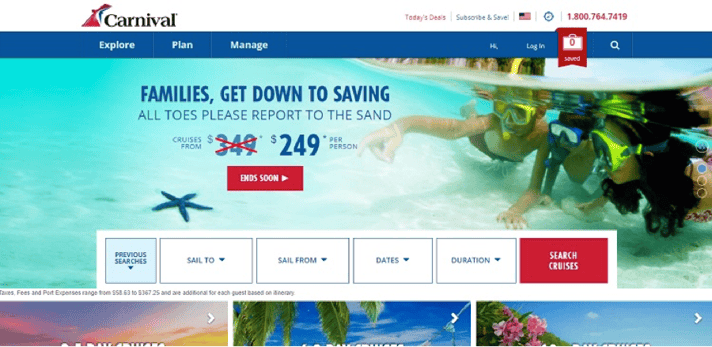At the top of the image, there is a white bar featuring the Carnival logo, which resembles a red boat stabilizer. To the right, the bar includes links for "Today's Deals," "Subscribe and Save," a U.S. flag presumably for language selection, a blue circle with indistinct details, and a phone number. Below this is a blue navigation bar with options for "Explore," "Plan," and "Manage," followed by "Log In" on the right. There is also a red ribbon icon with a suitcase and a zero, some unreadable text, a magnifying glass, and a text box for search functionality.

The main section of the image shows three people snorkeling underwater, captured at the terminator between air and water, giving a glimpse of the air above them. Overlaid text reads, "Families, get down to saving. All tows please report to the sand. Cruises from $349 [crossed out] $249 per person." 

At the bottom of the picture, there are options for "Previous Searches," "Sail To," "Sail From," "Heights," "Duration," and "Search Cruises." Below this section, three images in a row hint at tropical locations with blue skies, though they occupy less than a quarter of the height of the main image.